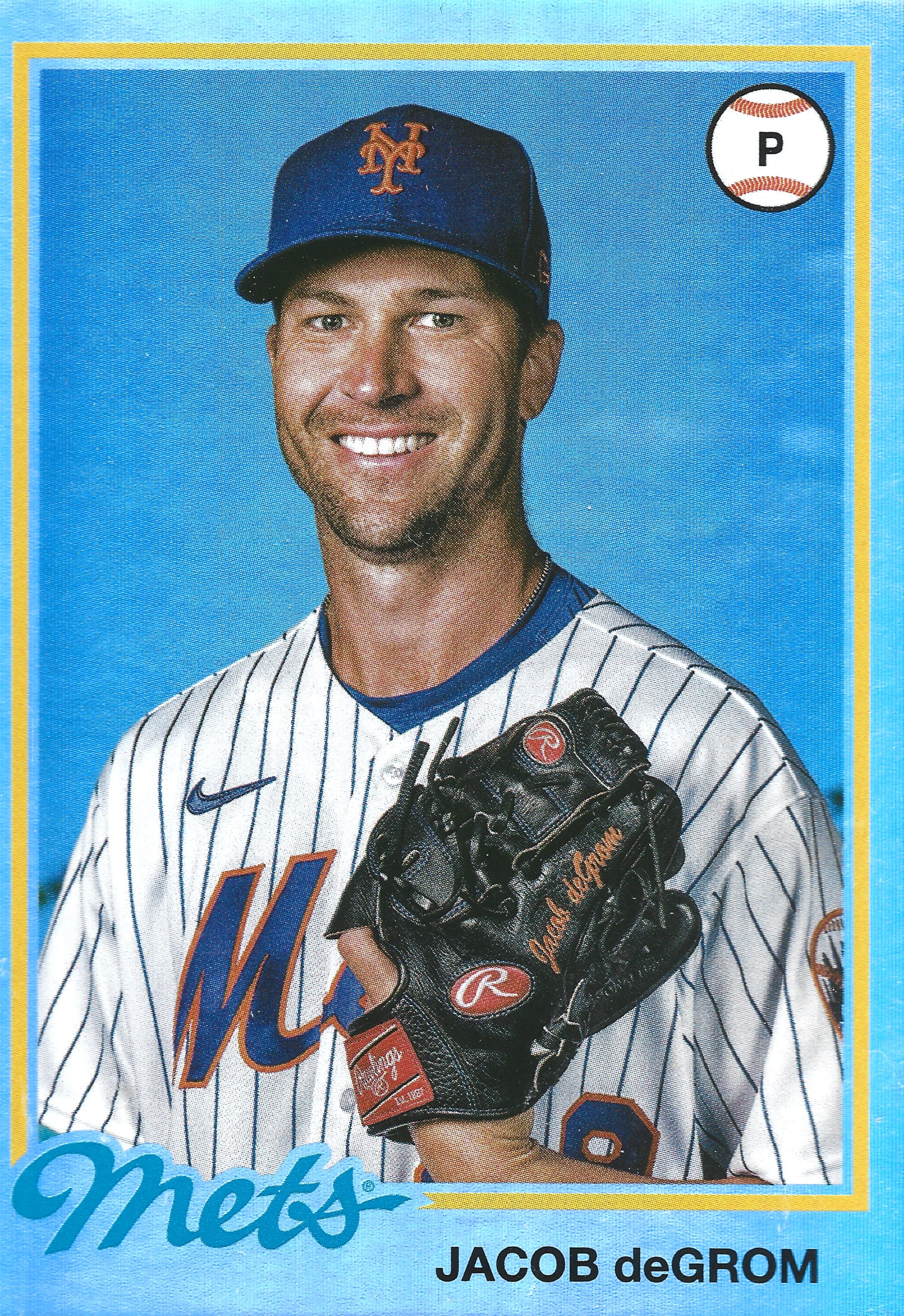The image is a baseball card featuring Jacob DeGrom, a player for the New York Mets. The card has a light blue frame with an additional thin yellow border. Within the frame, Jacob DeGrom is smiling, showing his top teeth, and wearing a blue hat with orange "NY" lettering, indicative of the Mets. His uniform is white with blue pinstripes, featuring the Mets logo in blue with an orange outline on the front, and a blue Nike swoosh above the logo. 

The background of the image is pixelated and blue, contributing to a grainy texture. DeGrom's left hand is holding a black catcher's mitt, displaying it prominently in front of him. The glove has some illegible writing at the top part, with "Jacob DeGrom" inscribed in black letters on a light blue background near the bottom right.

Additional details include the card having a white and blue outline accented by a yellow line, with a white baseball featuring red stitching and a black "P" at the top right corner. The bottom part of the card shows "Mets" written in blue cursive on a light blue background in the lower left corner, and "Jacob DeGrom" in black letters at the bottom right. The overall image is characterized by its pixelation and rough texture, giving it a distinct, detailed appearance.